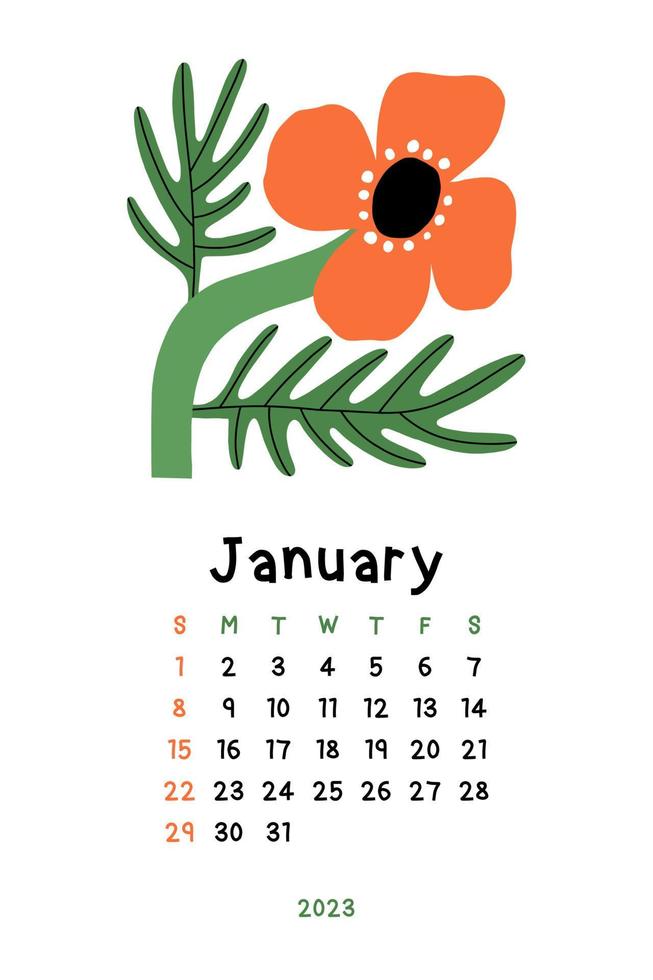This image is a digital scan of a calendar for January 2023, with a decorative illustration occupying the top portion. The illustration features a dark orange flower with four large petals radiating from a black center encircled by small white dots. The flower is anchored by a dark green, thick stem that curves slightly to the right, supporting two irregularly shaped, spiky leaves—one on either side of the stem. The calendar dates for January are laid out below the flower, with Sundays highlighted in red, other days' letters in green, and numbers in black. At the bottom, the year 2023 is written in green.